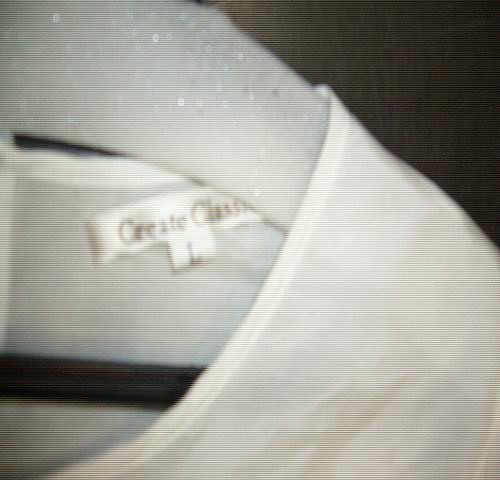The photograph depicts a close-up view of a coat hanger holding a white shirt or top. The image is slightly blurred or low-resolution, making the details somewhat indistinct. The shirt on the hanger is labeled "Creative Classic" with the size indicated as "L" on the inside near the collar. The shirt features a round collar with no pronounced neckline. The coat hanger itself is adorned with glitter on the top part, while the bottom straight section is black.